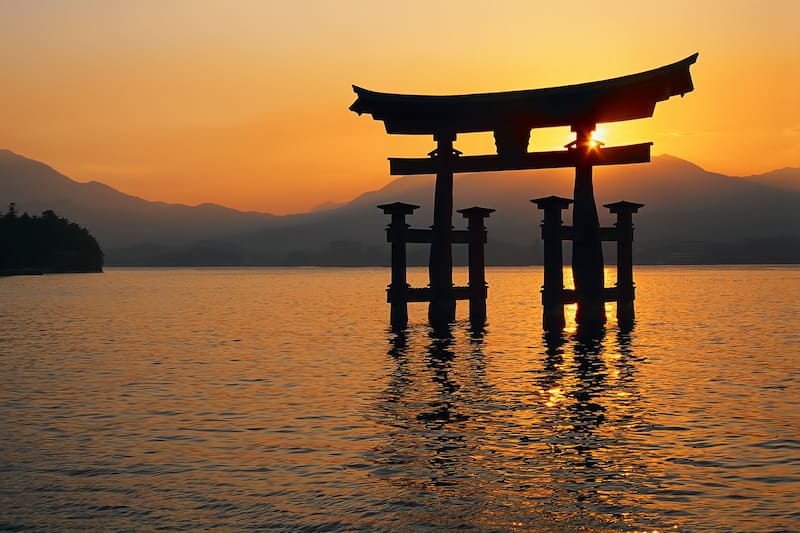The image is a richly detailed outdoor photograph captured during a sunset. Dominating the scene is a striking, silhouetted Japanese-style Shinto structure, reminiscent of an ancient temple arch, standing alone in the middle of a serene lake. This structure comprises two main vertical columns, supported by additional columns on either side, connected by a horizontal beam. On top of this beam rests a curved element, evoking the aesthetic of a traditional pagoda. The sun, a vibrant orange, sets just above the mountainous horizon, casting a golden hue across the sky and water. The water beneath the structure reflects this warm glow, mirroring the deep oranges and lighter yellows of the sky. The distant mountains stand grey against the colorful backdrop, adding to the tranquil yet majestic atmosphere of the scene. There is also a shadowy landmass covered in trees visible on the right, enhancing the depth of the landscape.